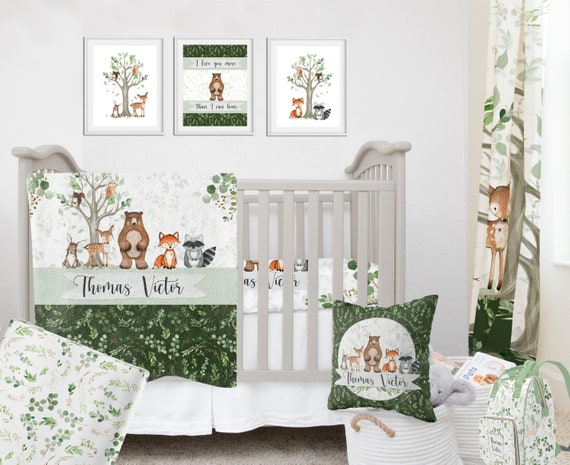This image captures a meticulously staged baby nursery with a serene woodland theme. The room features a backdrop of a white wall, adorned with three identically sized, white-framed pictures above a gray crib. Each picture contains charming forest scenes: a deer behind a tree with a yellow and brown bird, a bear, and a tree with a fox, raccoon, and additional birds. The crib itself is accessorized with a woodland-themed blanket draped over the rail, inscribed with "Thomas Victor" alongside images of a rabbit, deer, bear, fox, and raccoon. The bed's white bedding aligns with the room's color scheme, predominantly muted greens and whites. To the right of the crib, a curtain echoes the woodland design, as do various pillows scattered on the floor, one of which is green with a similar pattern. Books are tucked into a basket beneath the pillows, and a floral backpack is visible in the bottom right corner. The light tan carpeting and the overall coordinated decor suggest this could be an advertisement for a complete nursery ensemble, perfect for a new baby.